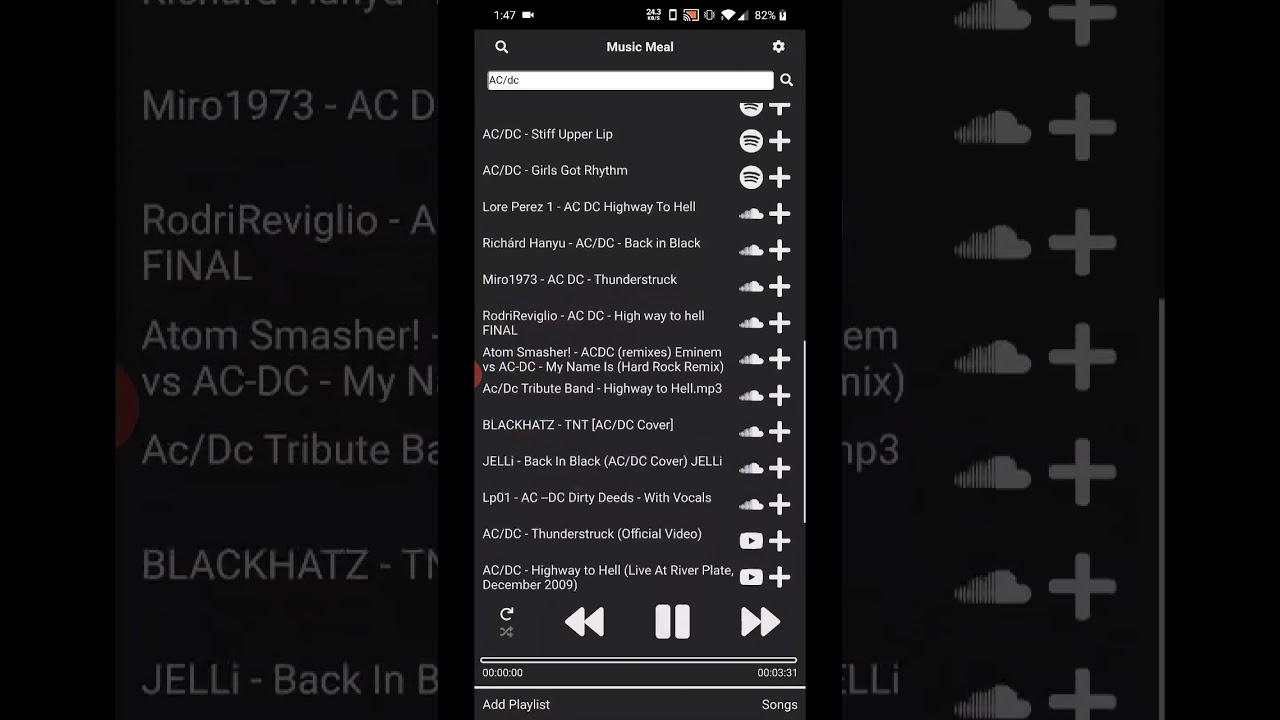This image is a detailed screenshot of a web page with a black background primarily displaying a music playlist interface. In the backdrop, there's a magnified, slightly grayed-out version of the list that serves as a visual element. The main content in the foreground is a section titled "Music Meal," which sits above a search box. The search box contains a partially obscured term, appearing to start with "AC," although the full text is not clear.

Directly below the search box is a list of approximately 10 different songs, each accompanied by several icons aligned to their right. Beneath this song list is a set of music control buttons: a forward-facing arrow with a rounded design, whose function is uncertain; followed by a rewind button, a pause button, and a fast-forward button. Further down the page, there is additional text and details that are too small to decipher from the screenshot.